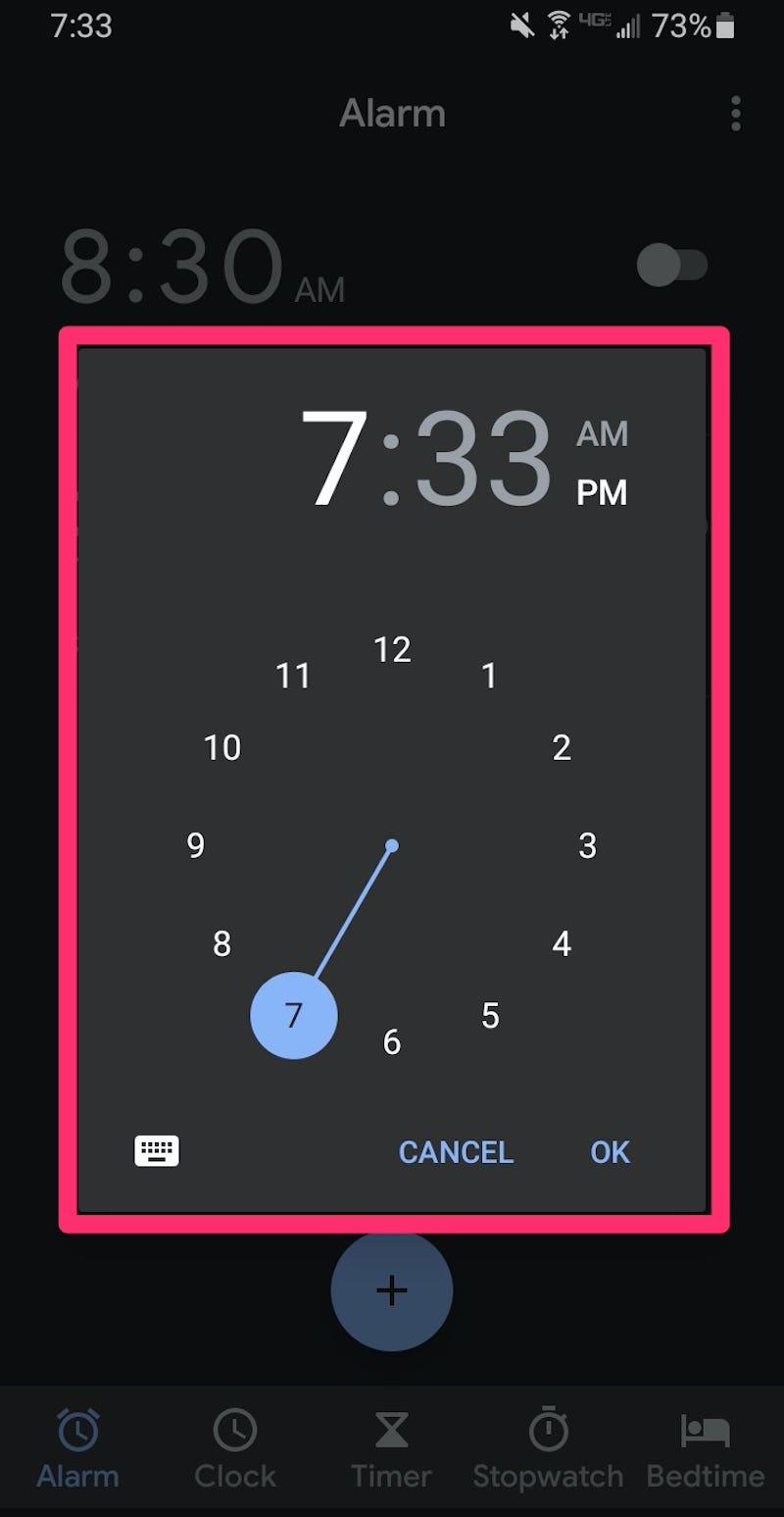This image is a screenshot of a mobile device's clock application interface. At the top left corner, the device's time is prominently displayed as 7:33 PM. On the top right corner, the status bar contains several icons including a mute icon, a Wi-Fi signal icon, and a network signal bar showing 3 out of 5 bars. Additionally, the battery level is visibly at 73%. Below this, an alarm is set for 7:33 PM, making the time and alarm synchronized. The bottom section of the image showcases tabs for various clock functions: Alarm, Clock, Timer, Stopwatch, and Bedtime. The overall color scheme of the interface includes white text and icons set against black backgrounds, with elements of red and blue highlighting specific features.